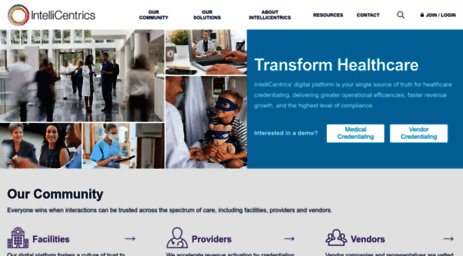**Detailed Website Description:**

The image under the "Websites" category features a compact and somewhat condensed webpage, making it challenging to read the finer details. At the top, there is a vibrant, multicolored circle with the text "IntelliCentrix" prominently displayed. Surrounding this logo are several dark blue menu categories running horizontally across the top of the page, though they are too small to decipher clearly. Distinguishably, one menu item labeled "Contact" and another "Login" can be identified, along with an icon of a magnifying glass likely representing a search function.

Beneath the navigation menu, a prominent picture depicts a bustling hospital hallway. In the foreground, a woman is dressed in a white lab coat, engaging in conversation with a man in scrubs. Another man, also in a white lab coat, is seen walking away and appears quite blurry. Adjacent to this scene, there's an additional image showing a compassionate doctor conversing with a child who is resting in a hospital bed. The child, wearing a blue mask, holds a teddy bear that is donned in a matching blue mask, emphasizing care and empathy.

Below these images, a teal blue box stands out with the bold text "Transform Healthcare." Directly underneath, it states, "Our community facilities, providers, vendors," reflecting the website’s commitment to comprehensive healthcare services.